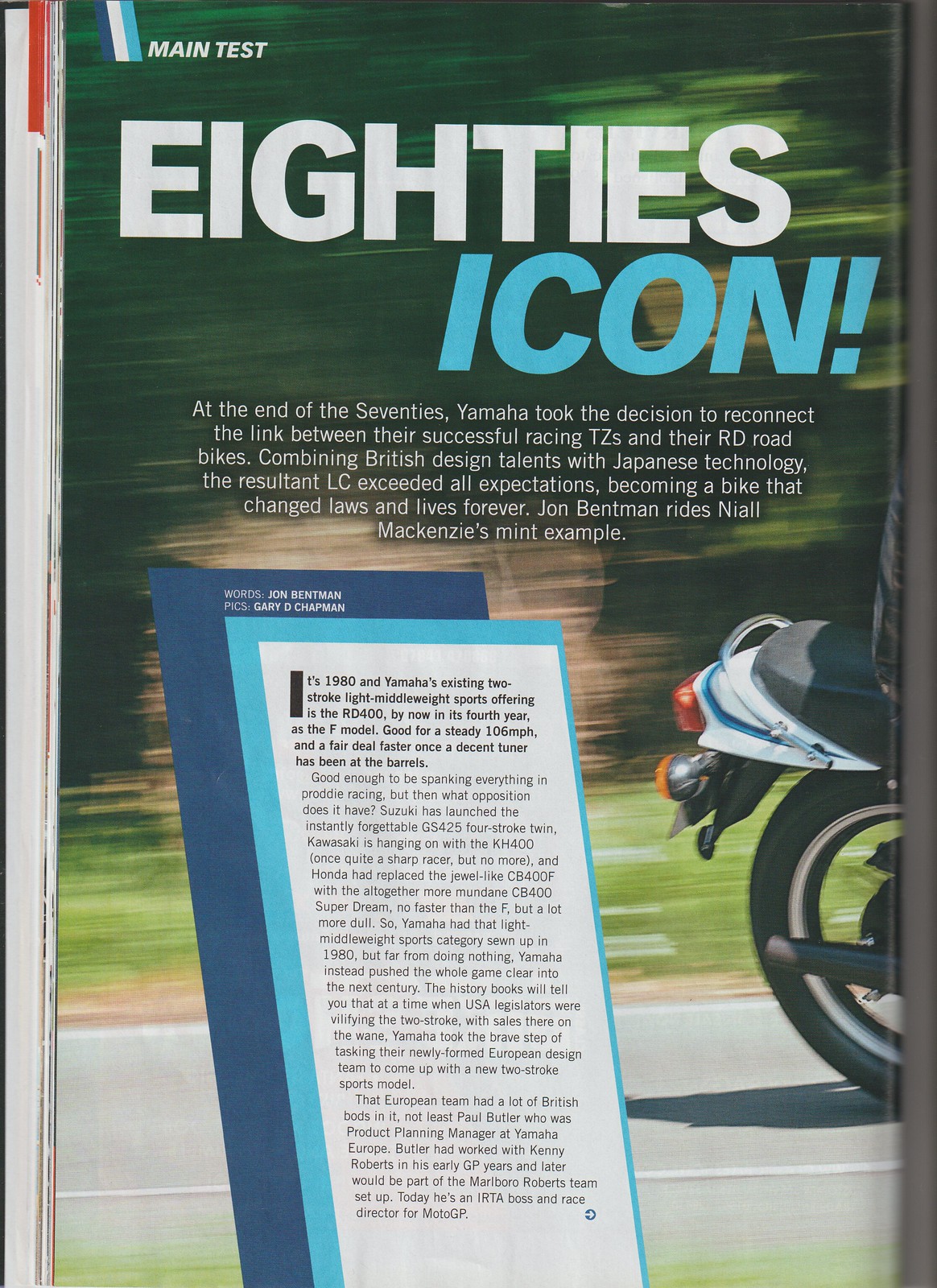The image appears to be a page from a magazine, prominently featuring a stylized greenish backdrop with smears of green at the top. The top-left of the page contains the text "main test" in small letters. Below this, in white, is the title "80s," and just beneath that, slightly to the right, is the word "icon" in a light blue color with an exclamation mark. The article reads: "At the end of the 70s, Yamaha took the decision to reconnect the link between their successful racing TZs and their RD road bikes, combining British design talents with Japanese technology. The resultant LC exceeded all expectations, becoming a bike that changed laws and lives forever. John Bentman rides Niall McKenzie's mint example." On the right side of the page is the tail end of a motorcycle. Additionally, there is a box of text with a turquoise border, which itself is outlined by a blue border. The colors present in the image include greens, grays, whites, blues, oranges, lighter blues, and lighter greens.